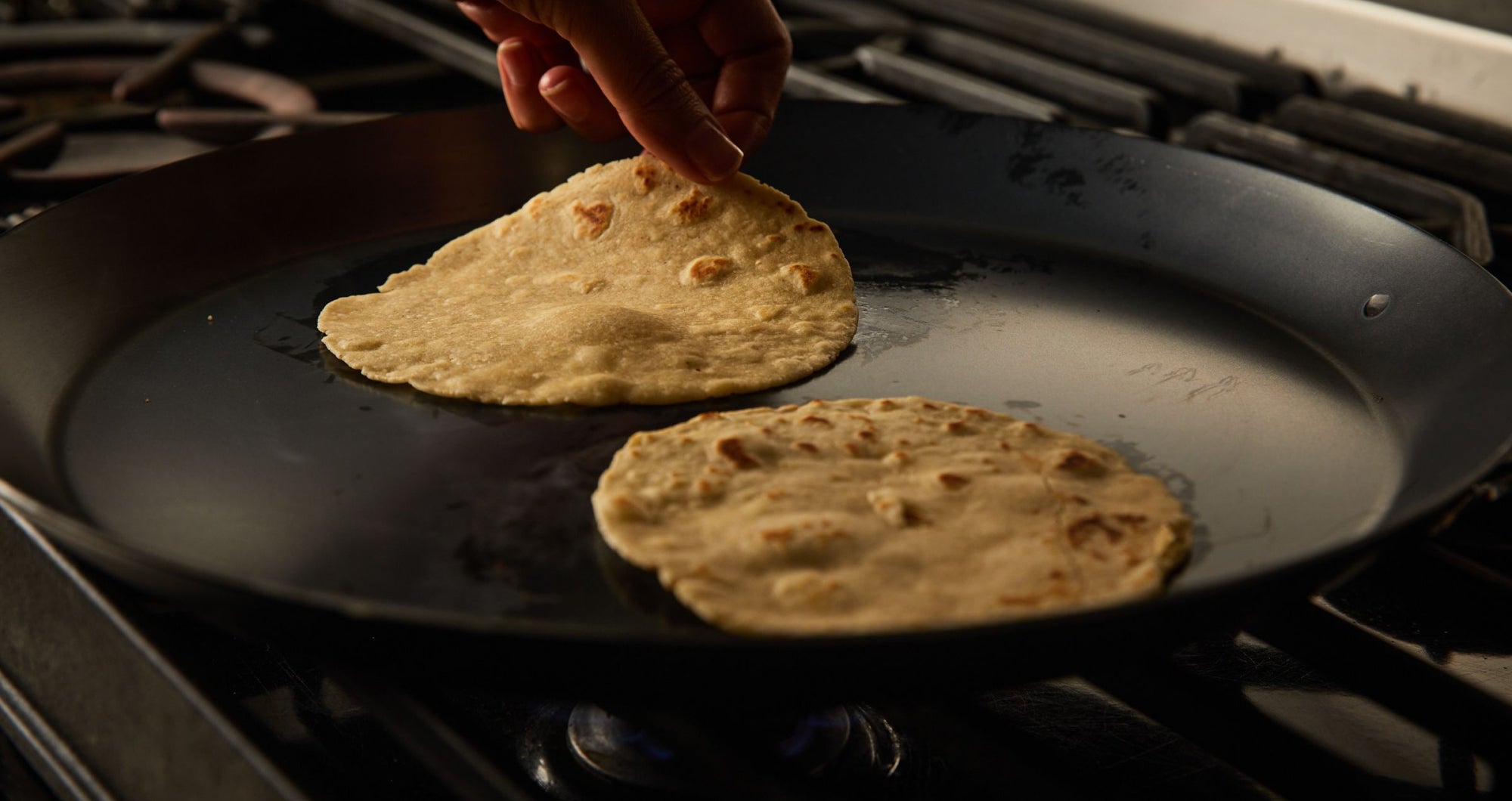In the close-up image, a left hand with a French manicure is seen lifting a toasted, hand-sized tortilla from a black skillet on a black stovetop. The scene is set in a kitchen, with a white frame visible in the background. The skillet is clean, holding two tortillas side-by-side, which are slightly burnt and bubbling. The stovetop appears to be a gas range with a metal grill at the front, providing context to the cooking atmosphere. The detailed focus on the hand and the tortillas highlights the process of making tortillas, capturing a precise, intimate moment in the kitchen.